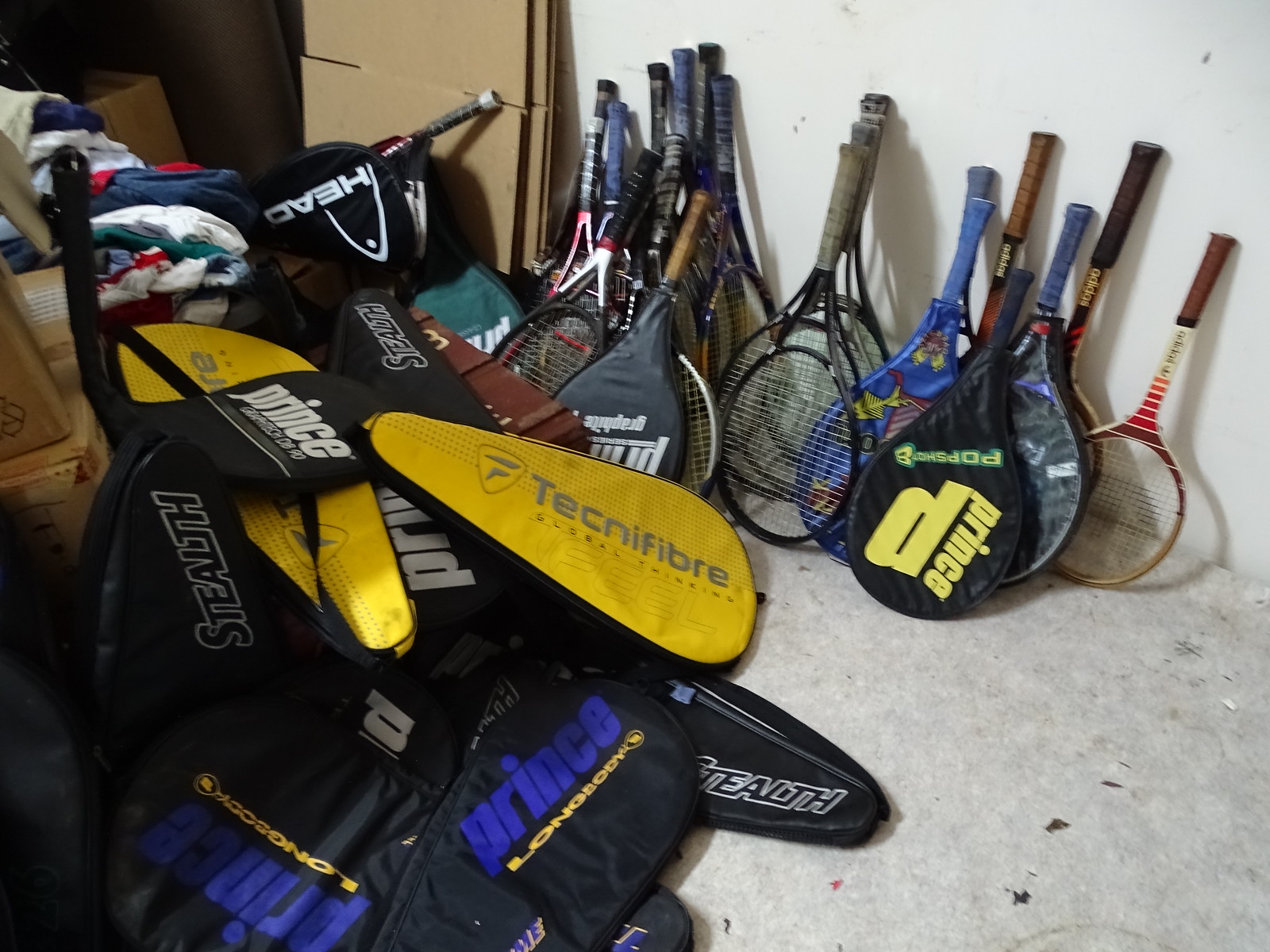This image captures a nondescript room that appears to serve as a storage space for sporting equipment, possibly linked to a gymnasium or tennis academy. The floor is concrete, and the walls are an unremarkable gray, further emphasizing the utilitarian nature of the space. Leaning against one side of the room, you can see around fifteen tennis rackets, their handles resting against the wall. The rackets vary in brands and colors, including Prince, Technofiber, Head, and Stealth, with some featuring retro designs and others in shades of blue and black. To the left, there is a disordered heap of tennis racket covers and a few cardboard boxes, adding to the cluttered appearance. The scene suggests a storeroom meant for communal use, possibly catering to visitors who may not have their own tennis equipment.